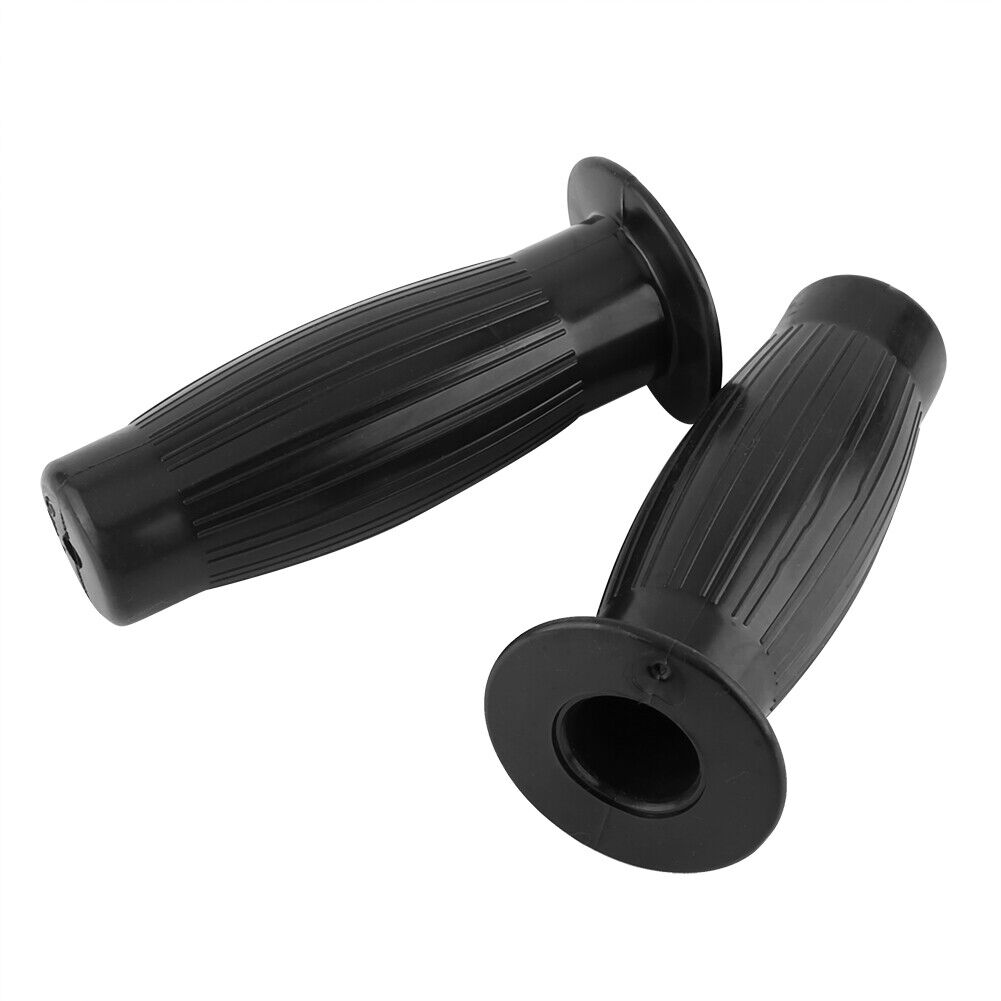This is a professional color photograph set against a completely white background, leaving the focus solely on two shiny, black cylindrical objects positioned horizontally next to each other. Each object features numerous grooves and lines, giving them a detailed texture. The bottom of each cylinder has a hole, creating a distinctive opening. Resembling hand grips for a bicycle, these black objects appear to have a stopper-like part at one end, similar to handlebar grips. Their precise material is unclear, with possibilities ranging from metal to plastic or rubber. Despite the ambiguity in their exact function, their sleek and reflective surface adds to the structured, yet minimalist aesthetic of the image.